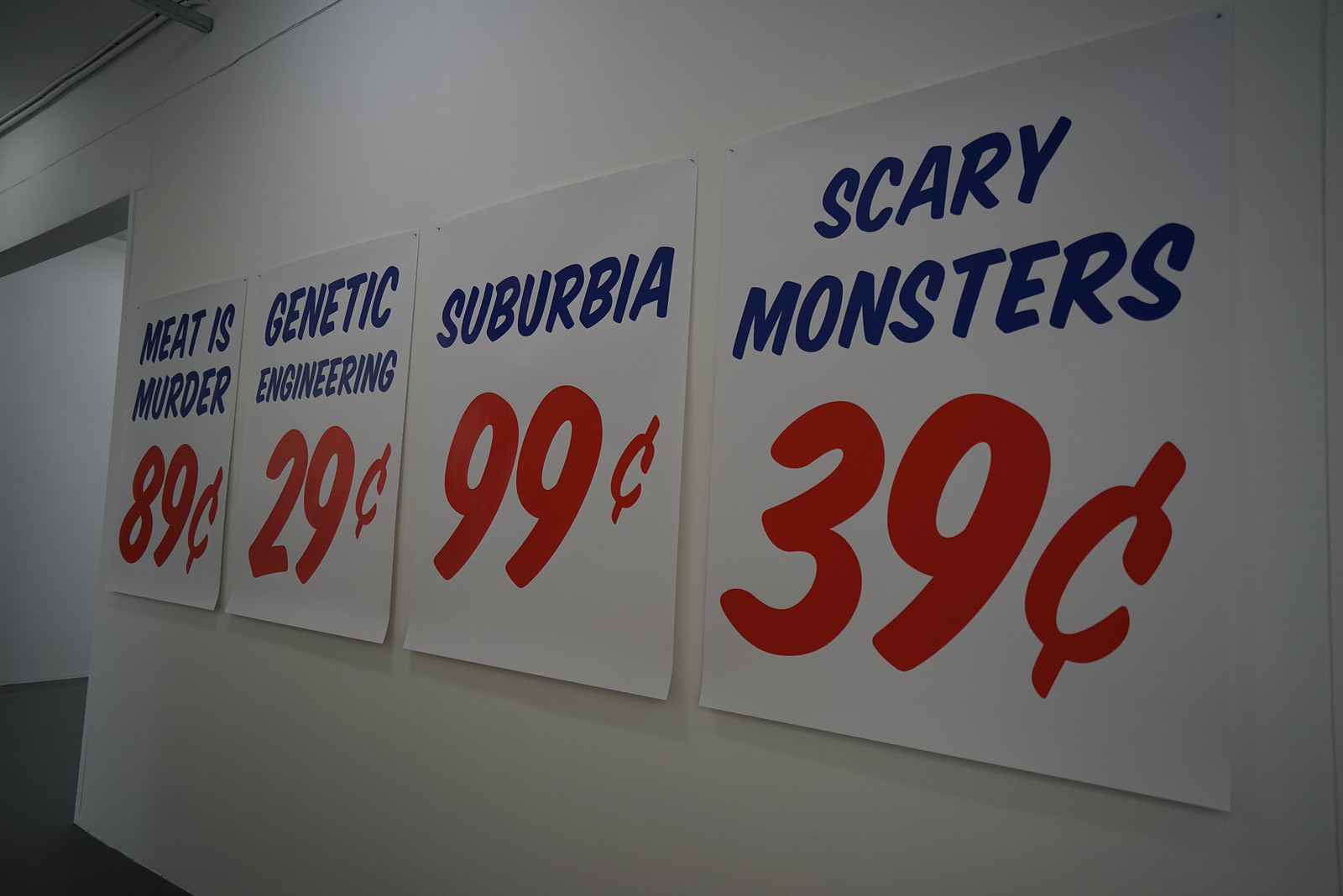In this intriguing image, a stark white wall serves as the canvas for four cryptic signs. Positioned along the wall, these signs feature bold statements, each paired with a price. The signs are crafted with white backgrounds, with the text rendered in a combination of red numbers and blue letters. On the far left side of the frame, a doorway discreetly appears. The first sign reads "Meat is murder" priced at $0.89. Moving rightward, the second sign declares "Genetic engineering" for $0.29. The third sign ominously labels "Suburbia" at $0.99. Closest to the right-hand edge, the final sign chillingly states "Scary monsters" for $0.39. The significance of these prices remains ambiguous, inviting viewers to further explore the context.